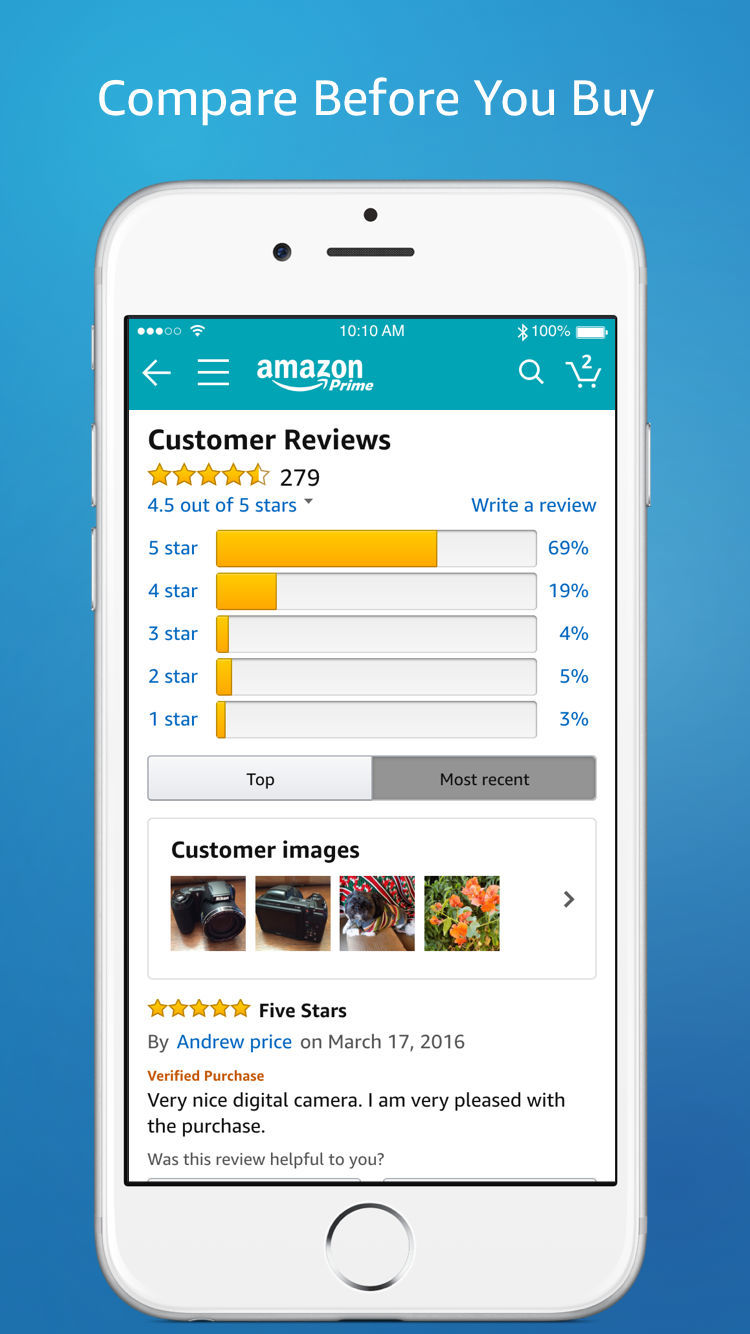This image showcases a circular blue and black graphic with the text "Compare Before You Buy" prominently displayed at the top. Below this graphic is a white smartphone, revealing its side buttons, top holes, and detailed interface display. The phone screen exhibits an Amazon Prime page interface. At the top of the screen, status indicators show full cell signal bars, Wi-Fi connectivity, 10:10 a.m. time, 100% battery charge, and Bluetooth enabled. Navigation icons such as a back arrow and a menu represented by three stacked lines are displayed alongside the Amazon Prime logo, a magnifying glass search icon, and a shopping cart indicating two items.

The phone's interface has a green-teal header and a white background. It features "Customer Reviews," showing a rating of 4.5 out of 5 stars based on 279 reviews. A detailed breakdown of the reviews is provided with the following distributions: 69% five-star, 19% four-star, 4% three-star, 5% two-star, and 3% one-star ratings. Below this breakdown are interactive elements: a white button with black text labeled "Top" and a gray button with black text labeled "Most Recent."

Additionally, the page features a section titled "Customer Images," displaying four images. Underneath is a specific review: "Five stars by Andrew Price on March 17, 2016 - Verified Purchaser. A very nice digital camera, I'm very pleased with the purchase." There is an option asking if the review was helpful, presented in gray text.